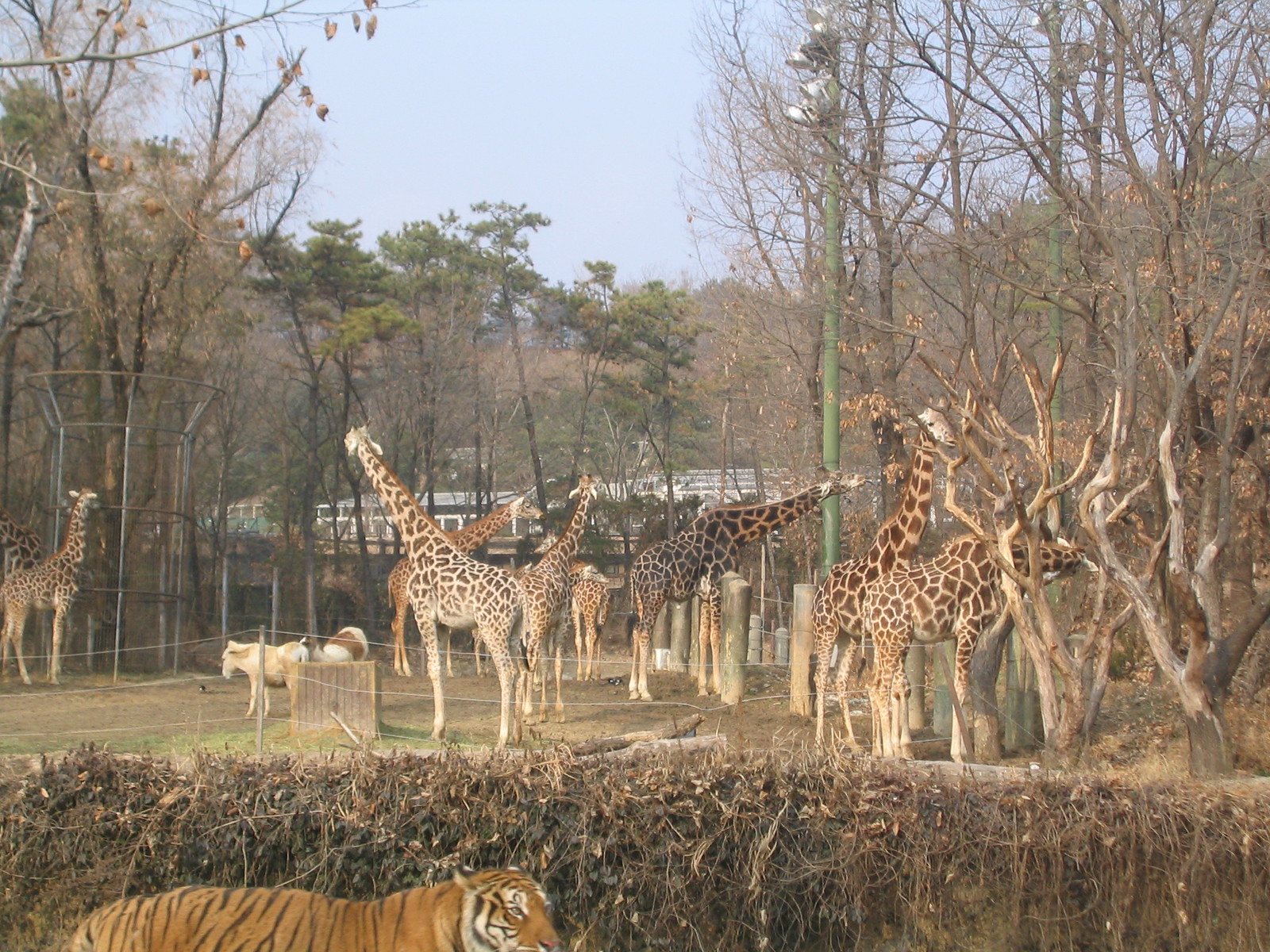This photograph captures a zoo enclosure during winter, featuring a variety of animals and intricate details of their habitat. In the foreground, a partially visible tiger is separated by a rustic, vine-covered retaining wall and wire fence. The tiger occupies the lower left portion of the image. Behind the brush wall, there is an expansive enclosure containing eight giraffes and two goats interspersed throughout the frame. Sparse trees with few leaves, indicating the winter season, populate the enclosure. The habitat is delineated by wooden posts with wires strung between them. In the far background, there are structures resembling a building with numerous windows, possibly a tram or buses. This setting suggests a zoo or safari park, likely in a region where enclosures are designed in close proximity to mimic natural habitats. The sky above is clear, further emphasizing the wintry, open environment.